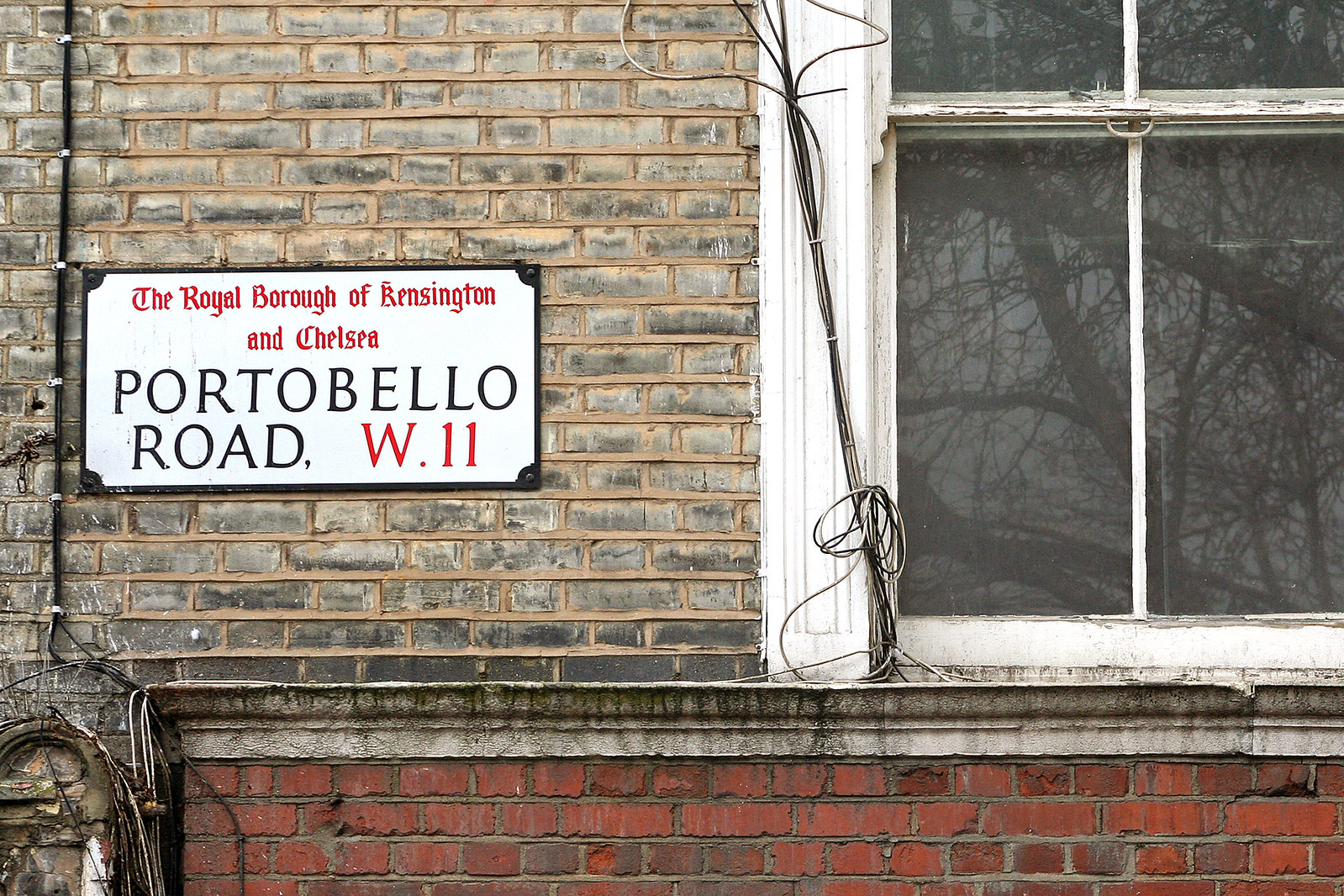This is a detailed image of a brick building featuring a two-toned brick wall. The upper section of the wall is constructed with gray bricks and tan mortar, while the lower section consists of red bricks with gray mortar. A white framed window is situated to the right of the gray bricks, with some wiring extending down from it, and a window sill rests above the red brick section. Adjacent to the window, there is a sign affixed to the building. The sign is white, trimmed in red text, and reads: "The Royal Borough of Kensington and Chelsea" in Old English script and "Portobello Road W11" in capital letters below. This combination of architectural features and detailed signage showcases both the historical and urban elements of the building's facade.